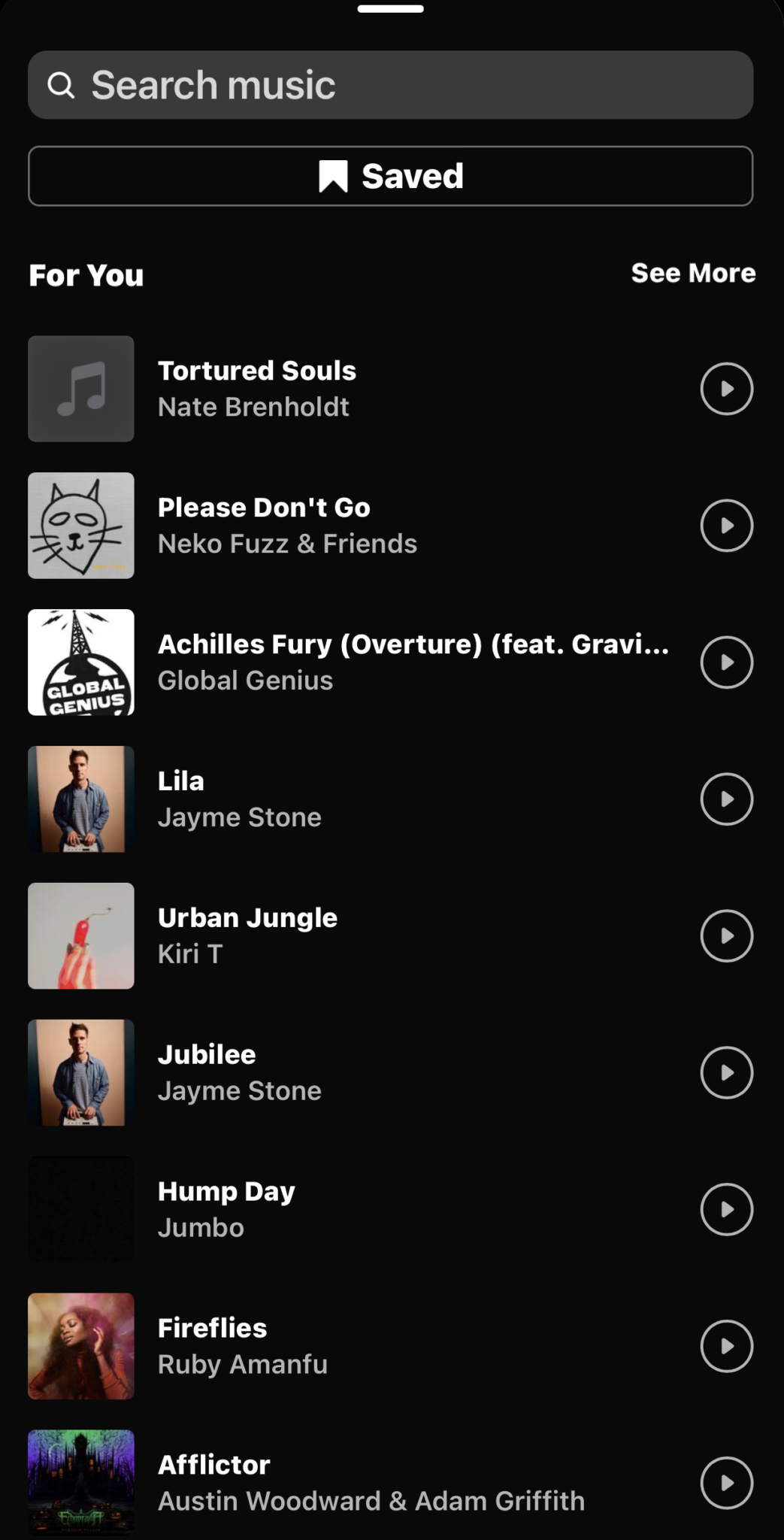The image depicts a screenshot of a music application featuring a curated playlist. The playlist includes nine distinct songs, each listed with their respective artist names. The entries in the list are:

1. "Urban Jungle" by Artist Unknown
2. "Hump Day" by Jumbo
3. "Fireflies" by Ruby and Menfu
4. "Tortured Souls" by Nate Brenholt
5. "Please Don’t Go" by Nico Fuzz and Friends

At the top of the screen, there is a search bar labeled "Search music," allowing users to find specific tracks or artists within the application. Directly below the search bar is a prominently displayed, elongated save button, matching the search bar in size and facilitating the saving of the playlist or individual tracks.

The interface features a sleek black background with white text, ensuring high contrast and readability. This music application is presented on a mobile phone, showcasing a user-friendly and visually appealing format for on-the-go music streaming and playlist management.